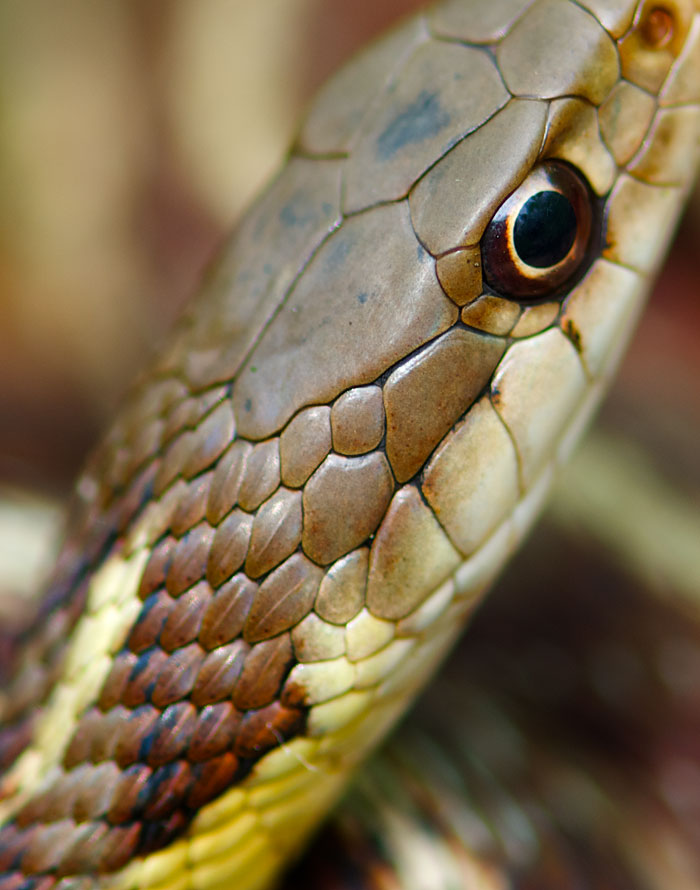This is an extremely detailed close-up photograph of a snake, focusing predominantly on its head and part of its neck. The top of its head is light brown with larger, irregular scales that resemble paving stones. The underside is cream or white, with a narrow stripe extending down its neck. The rest of its body features a mix of brown shades, with some of the scales appearing darker, and others lighter, arranged in small, uniform patterns. There are also at least two different shapes of brown diamonds along its back. The snake's eyes are particularly captivating, with a black pupil encircled by a bright copper or brown ring and a narrow, almost fiery white ring around the pupil, giving it an intense look. The head has a very flat top, and though the exact shape isn't clear, it seems well-defined. The snake's coloration transitions from its coppery head to more intricate brown and black scales as the body extends out of focus in the background.